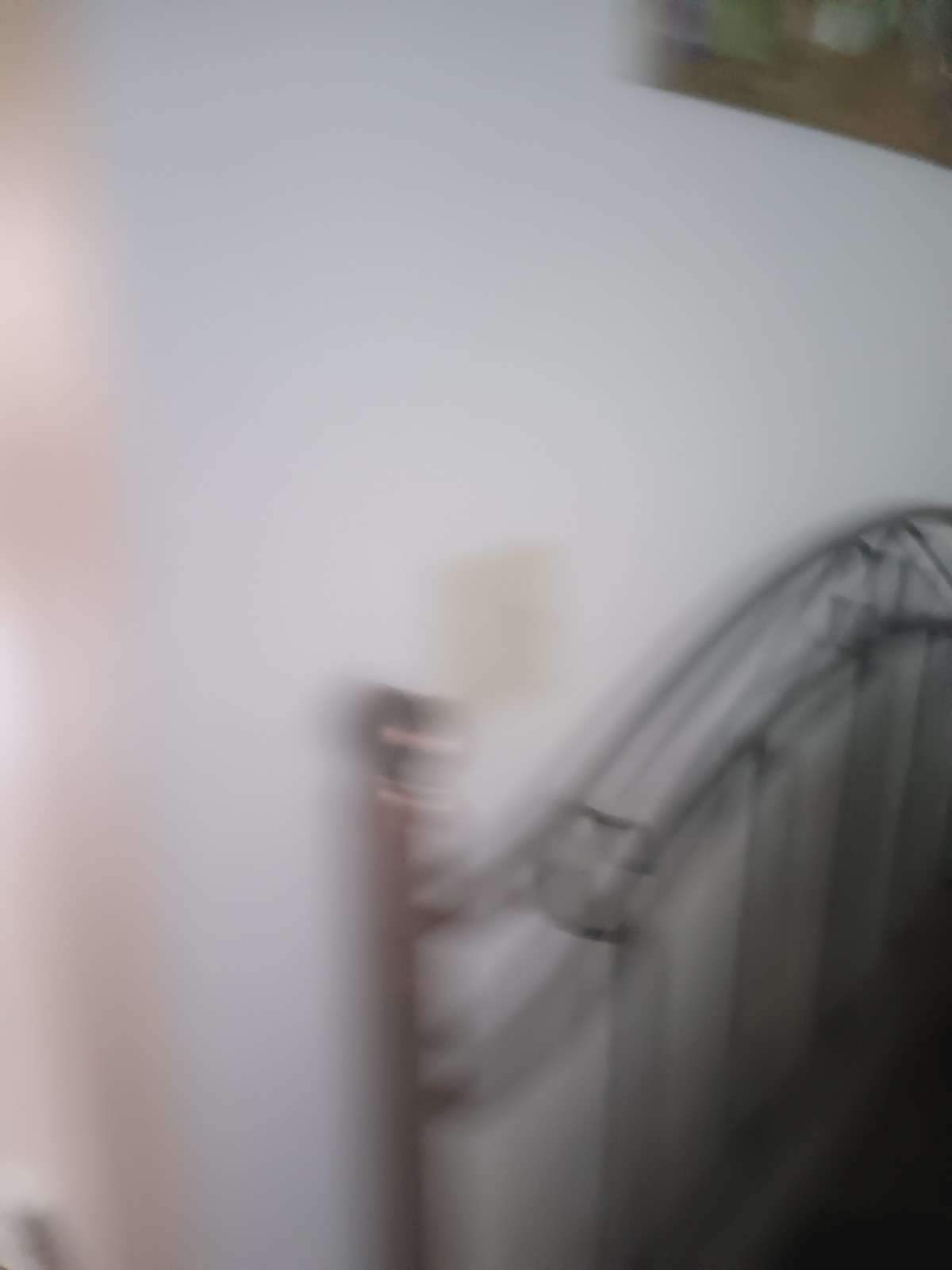In this image, a large brass headboard is the central focus. Though the picture is very blurry, the design of the headboard is discernible, featuring an intricate curve with two sections of metal arching gracefully. The headboard has four spindles, with one visible post that is topped by a decorative finial. Set against a white wall, the headboard highlights a noticeable discoloration stain on the wall behind it. The lower portion of the image is obscured by darkness, making it difficult to see anything clearly in front of the headboard. In the lower left corner, there's a black object whose shape and function are unclear. Above the bedpost, a brown-framed picture hangs on the wall, though the details within the frame remain indiscernible due to the image's blurriness.